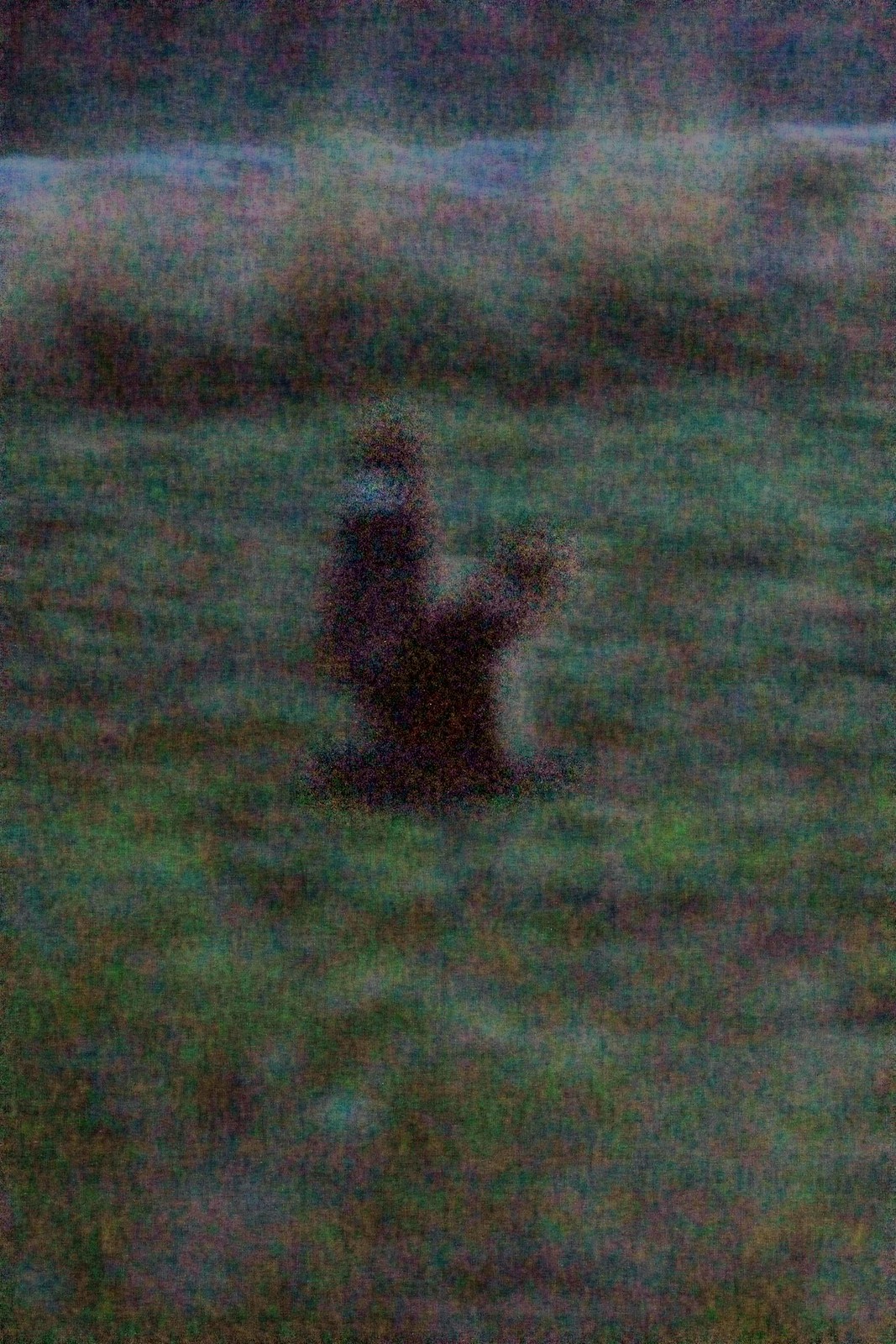The image depicts a very grainy and blurry scene that resembles an artwork more than a photograph. In the foreground, a bird in flight dominates the composition, but its details are obscured by the poor quality of the image. The bird's silhouette is visible, though it's unclear whether its dark appearance is due to its actual coloration or the fact that the photo seems to have been taken at night. The bird's motion adds to the overall blurriness, giving an impression of movement.

The background transitions from a grassy area with patches that suggest dirt or marshland, leading upwards to an indistinct mass of foliage. The vegetation presents itself in a spread of blotchy colors including green, brown, purple, and blue, blending chaotically due to the graininess. Beyond the foliage, there appears to be a dark surface that might be water or another indistinguishable landscape feature—its color shifting between blue and black.

In the middle of the image stand two ambiguous outlines that could be animals, discernable by their dark coats and shapes. There is also a suggestion of another animal-like figure, thought to resemble a squirrel, with a dark brown body and a whiter underbelly. However, the blurriness of the image leaves these supposed animals' identities up to interpretation.